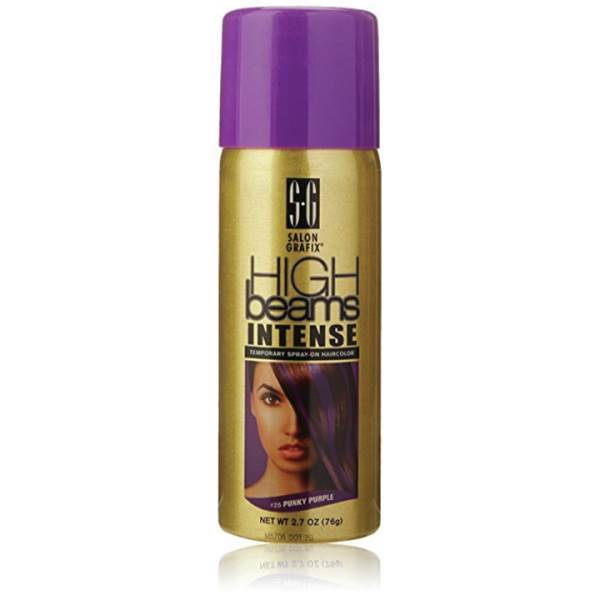This image depicts a beauty product designed for temporary hair coloring. Set against a white background, the central focus is a cylindrical canister in a striking gold color with a purple cap. The brand name "SG" is prominently displayed within a black box at the top of the can, followed by "Salon Graphics" in black text. Below this, in larger black letters, it reads "High Beams Intense." Further down, inside another black box with white text, it states "Temporary Spray on Hair Color."

Just below the textual information, there is a photo of a model with tanned skin, intense red lips, and auburn hair highlighted with streaks of purple. Her hair partially covers her left eye while she gazes intently into the camera with her right eye. Beneath her image, the text "25 Punky Purple" is displayed in white letters over a purple swirly background. Further down, the can provides additional details in black text, indicating a net weight of 2.7 ounces (76 grams). The reflection of the bottom part of the can is visible against the white backdrop, adding a touch of realism to the sterile, product-focused setup.